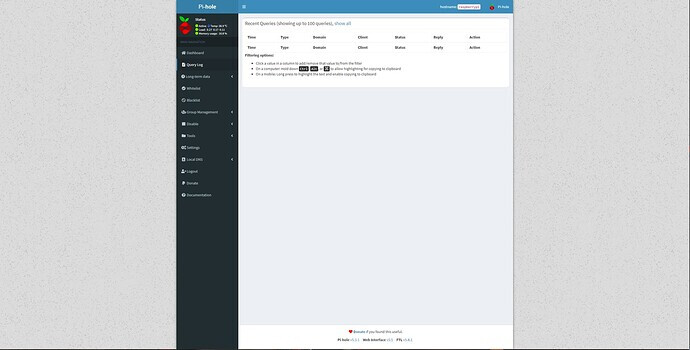This image showcases a website interface, categorized under "Websites," featuring a distinct layout and color scheme. Dominating the top portion of the interface is a blue navigation bar with white lettering that begins with the letter "P," though the exact text remains illegible. Positioned on the right side of this bar is a small search box.

Below the blue bar, on the left-hand side, there is a red fruit icon that appears to be either a strawberry or an apple, complete with green leaves. Adjacent to this icon is a vertical menu extending down the left side of the interface, comprising 13 distinct options, though the specific text of these menu items cannot be discerned.

To the right of the vertical menu, a white content box spans most of the remaining space. At the top of this box is a sentence, presumably providing context or a heading, followed by a grid layout featuring seven columns and two rows beneath each. Due to the small size of the text, the content within this grid remains unreadable.